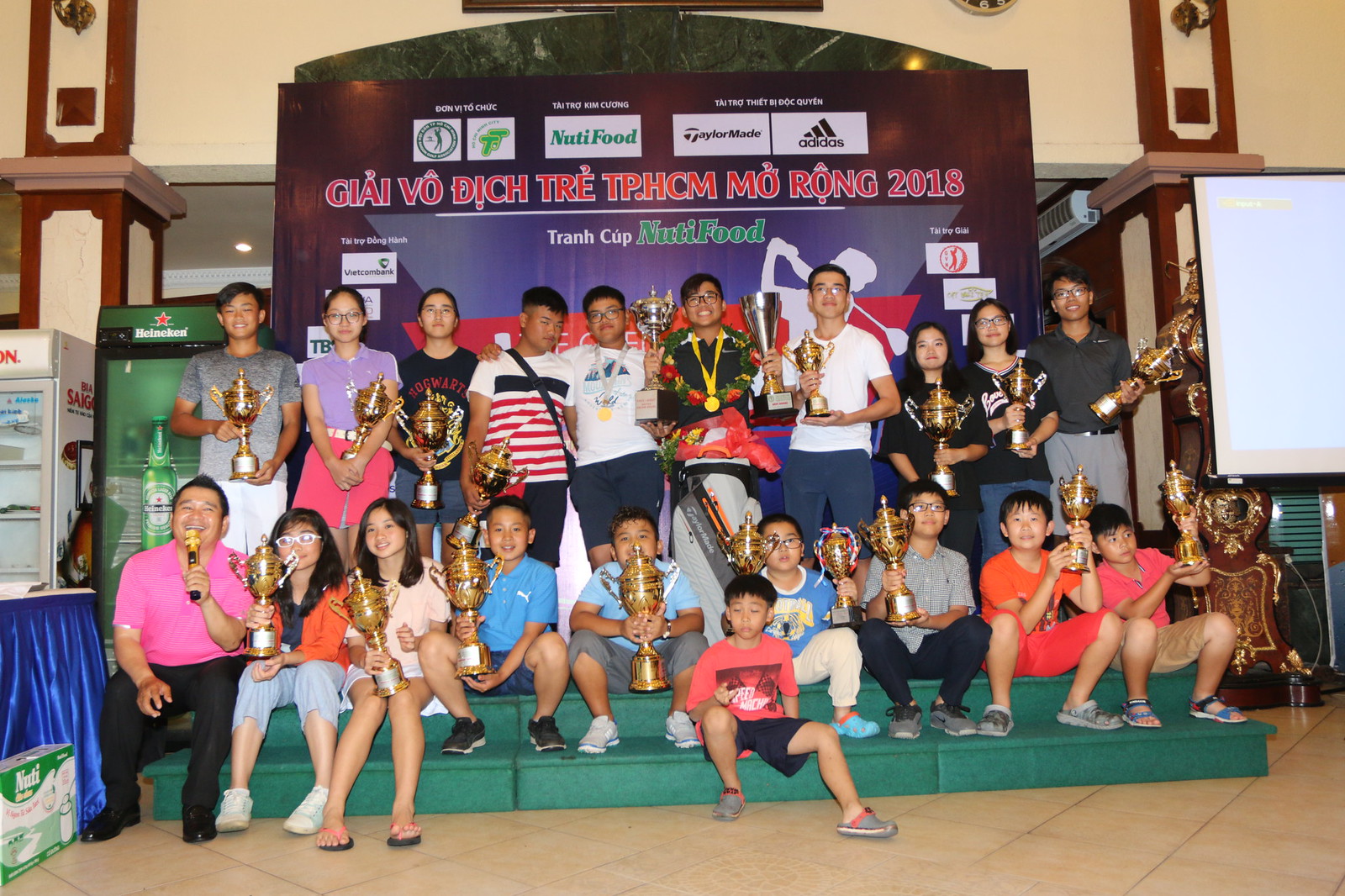The image depicts a vibrant scene featuring a diverse group of children, aged approximately five to ten, who have recently won a contest, possibly the "Tron Cup." Set within an indoor environment characterized by beige walls and tile floors, the children are assembled on green steps, with one row sitting and another standing behind them. Each child proudly holds a shiny, goldish-bronze trophy adorned with white elements. The children are dressed in various colors and styles, including red, green, blue, shorts, pants, t-shirts, and long sleeves, reflecting a lively mix of attire. Notably, there is an elderly man in a pink polo shirt on the left side of the image, holding a trophy to his mouth. A colorful sign with Vietnamese writing, advertisements—including one for Adidas—and a table with a blue cloth and a large screen in the right-hand corner of the room further detail the backdrop. The scene exudes a celebratory atmosphere showcasing the children's achievement in winning the contest.